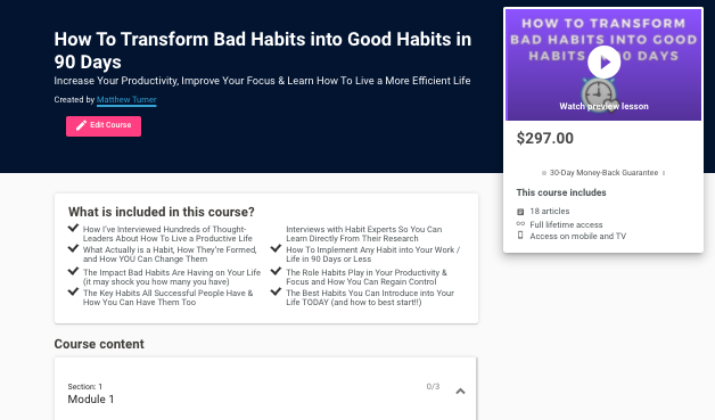**Course Overview: How to Transform Bad Habits into Good Habits in 90 Days**

**Instructor:** Matthew Turner

**Description:**
This comprehensive course, designed by Matthew Turner, aims to help you transform bad habits into good ones within 90 days. The course promises to increase productivity, improve focus, and teach strategies for a more efficient life. The main banner is blue with underlined text and features a red "Edit Course" button on a black horizontal rectangle. A white rectangle protrudes from the top right, displaying a purple background with a play button labeled "Watch Preview Lesson."

**Course Cost:** $297  
**Money-Back Guarantee:** 30 days

**Course Features:**
- 18 articles
- Full lifetime access
- Accessibility on mobile and TV

**Curriculum Highlights:**
- Insights from interviews with hundreds of thought leaders on productivity
- Detailed exploration of habits, their formation, and strategies for change
- Analysis of the impact of bad habits on your life
- Key habits of successful people and how to adopt them
- Exclusive interviews with habit experts to provide evidence-based learning

Embrace the opportunity to overhaul your habits and enhance your daily efficiency with this expertly crafted course by Matthew Turner.